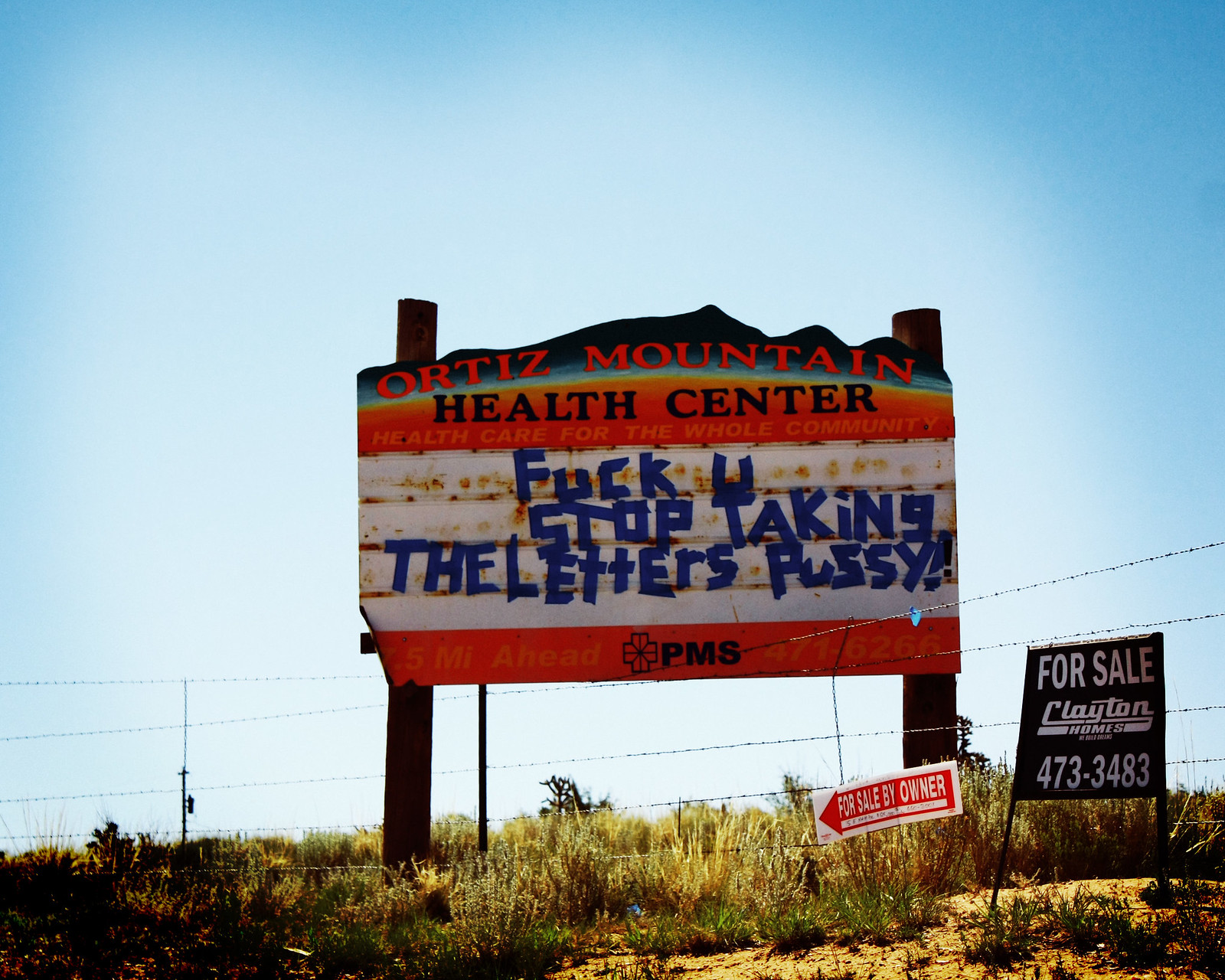In this daytime, outdoor photograph, under clear blue skies, we see a cluster of signs on a grassy, somewhat barren terrain that resembles a desert landscape. The main focus is a vintage, rectangular sign with a mountain-shaped top, reading "Ortiz Mountain Health Center" in orange letters on a green background, transitioning to blue letters on an orange background for the lower part of the text. Below this, the sign has a white segment with blue duct-tape graffiti stating "FUCK YOU, STOP TAKING THE LETTERS, PUSSY!" Beneath this, on a red borderline, the acronym "PMS" is written beside a cross flower symbol. To the right of this main sign, a smaller blue For Sale sign reads "Clayton Homes, 4733483" in white letters, secured with two stakes. Adjacent to this sign is another white "For Sale By Owner" sign with a red arrow. A barbed wire fence intersects the scene, adding to the rugged, uncultivated ambiance.